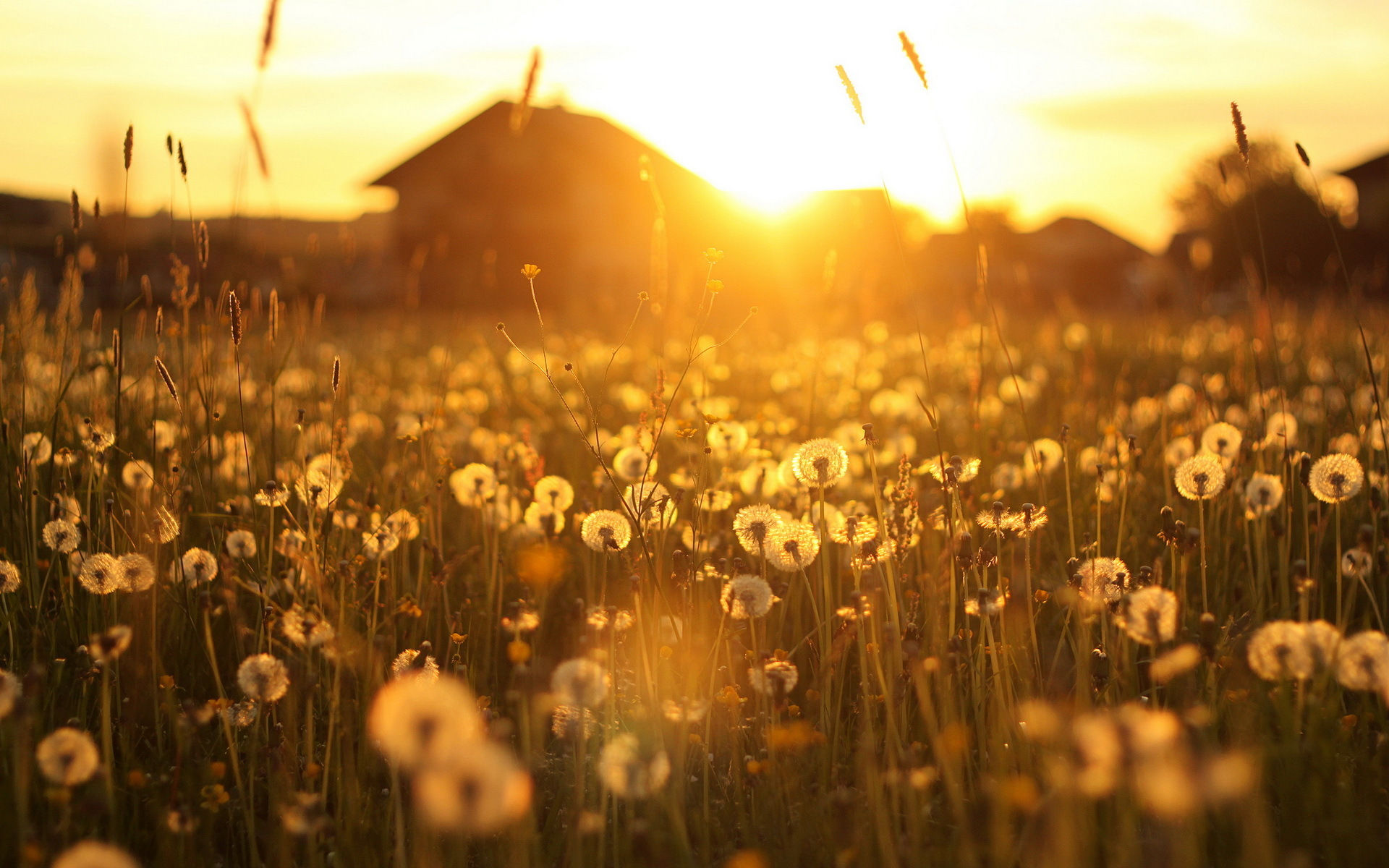This outdoor photograph, taken during either early morning or late afternoon, captures a tranquil field of tall milkweed dandelions bathed in a golden sunset. The image, roughly six inches wide and three inches tall, is dominated by warm yellow and brown hues, giving it a sepia-like tone. In the foreground, the dandelions and various grasses are in focus, creating a sense of being immersed in the field. The blurred background features several buildings, possibly houses or barns, partially obscured by the bright, low-hanging sun near the upper center of the horizon. This serene scene is suffused with the soft, warm light of the setting sun, highlighting the natural beauty and slightly untamed character of the field.